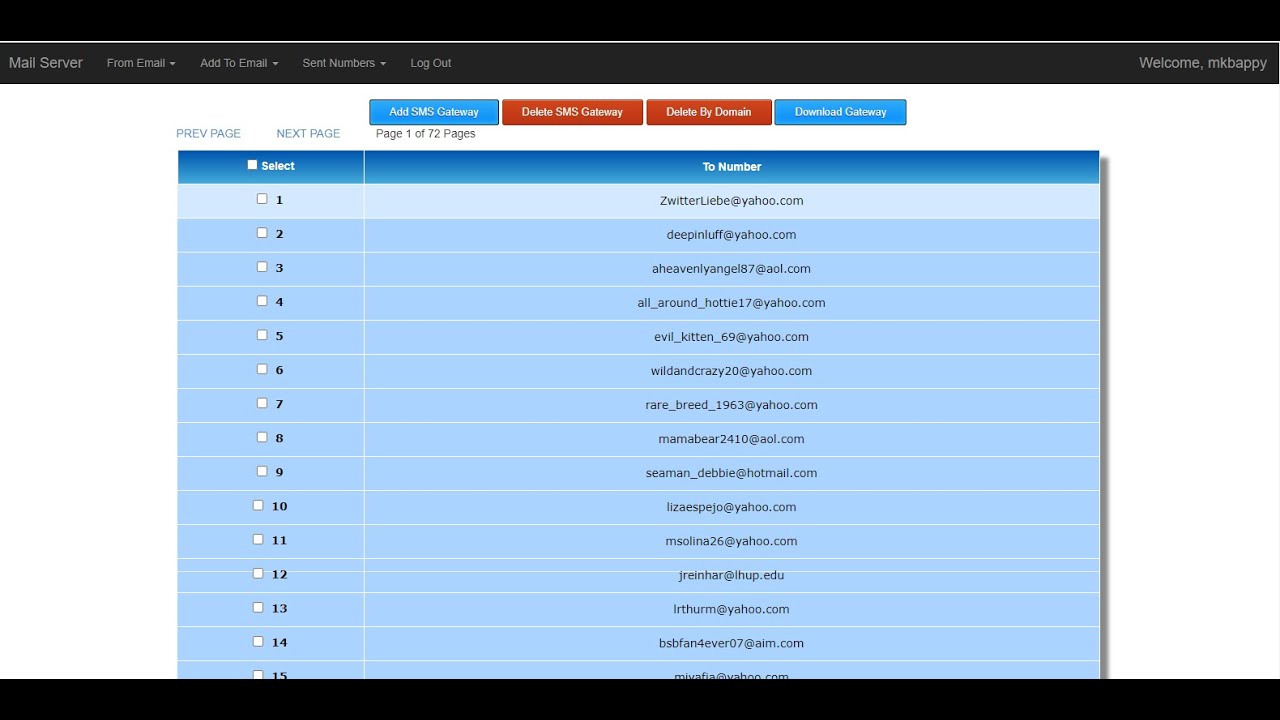The webpage displayed is a mail server dashboard. At the top, there's a black navigation bar with the title "Mail Server" prominently displayed. This bar contains various options such as "From Email," "Add to Email," "Sent Numbers," and a "Logout" button for user accessibility.

Just below, several categories and actions are organized, highlighted by blue buttons labeled "Add SMS Gateway," "Delete SMS Gateway," "Delete by Domain," and "Download Gateway," indicative of advanced SMS and email management functionalities.

A pagination section is present, depicting navigation options with "Previous Page" and "Next Page" buttons in blue, accompanied by a note stating the current view is "Page 1 of 72 pages." This confirms that the user can navigate through a substantial list of entries.

The main content area is a comprehensive list of email addresses, numbered 1 to 15 on the first page. Each entry includes a checkbox for selection, with an option to select all entries at the top. A specific example from the list includes addresses like "switterlieb@yahoo.com" and "deepinluff@yahoo.com," showcasing a variety of email contacts.

Additionally, a greeting on the page reads "Welcome mkbapi," indicating the logged-in user’s username. This list appears to facilitate the management and editing of email recipients, emphasizing an efficient, large-scale email distribution capability.